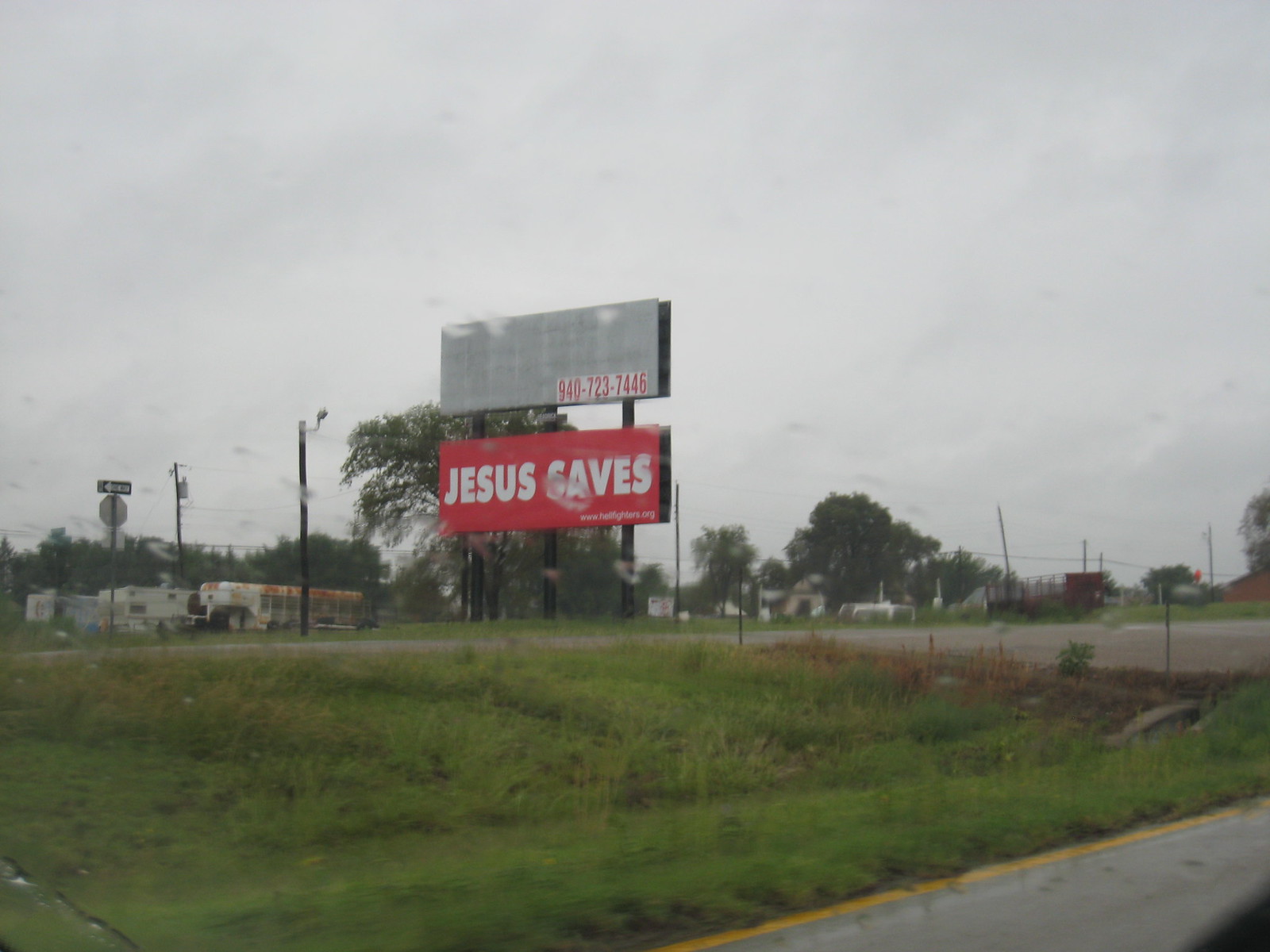The image captures a roadside scene taken from a moving vehicle. The main focus is on two large billboards positioned one above the other in the distance. The billboards, standing at least as tall as a large lamppost, dominate the background. The upper billboard has a simple grey background featuring a phone number, "940-723-7446," in bold red font. Directly below it, the second billboard is entirely red with the phrase "Jesus Saves" prominently displayed in white letters. Beneath these words, there is a web address that isn’t fully legible. Both billboards are supported by three massive pillars.

In the foreground, the image includes part of the road marked by a yellow line, indicating it's captured from a moving car. Following the road, there's a stretch of grassy area leading to another expanse of tarmac. Beyond this, another patch of grass and a scattering of trees come into view. There is a Shell gas station visible further in the background. Additional elements include some road signs, one resembling a stop sign, although we can only see the back of it. The prominent focus remains on the billboards towering above the scenery, directing attention to the message "Jesus Saves" and the phone number above it.